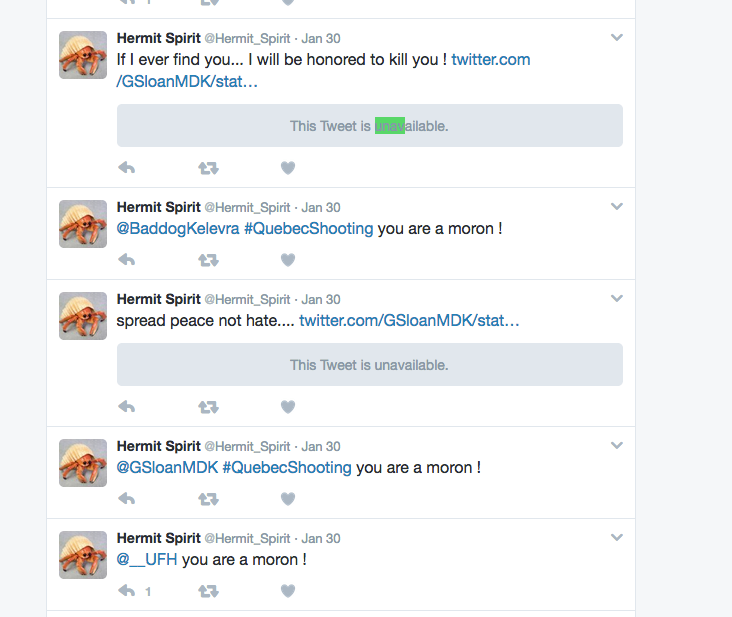This image is a screenshot of several tweets from the social media platform X, previously known as Twitter. Based on the content of the tweets, it likely dates back to when the platform was still referred to as Twitter, as indicated by the "Twitter.com" URL in one of the posts.

The prominent user in these tweets is @Hermit_Spirit, whose profile thumbnail features a bright orange hermit crab in its shell. The tweets are from January 30th and show a pattern of aggressive and confrontational language.

1. The first tweet reads: "If I ever find you... I will be honored to kill you!" followed by a broken URL link (Twitter.com/GSLOANMDK/stat…). This tweet is marked as unavailable.

2. The second visible tweet from @Hermit_Spirit is a reply to another user, @bad_dog_kill_livra, with the hashtag #QuebecShooting. It bluntly states: "You are a moron!" This tweet is also dated January 30th.

3. The third tweet from the same user promotes a message of peace but seems conflicting in context. It reads: "Spread peace not hate..." followed by another broken URL (Twitter.com/GSLOANMDK/stat…), which is again unavailable.

4. The fourth tweet is a repeat of the second, addressing @GSLOANMDK directly with the #QuebecShooting hashtag and the statement: "You are a moron!"

5. The fifth tweet, similarly aggressive in tone, is directed at @UFH: "You are a moron!"

The interface shows the typical Twitter interaction buttons for replies (symbolized by arrows), retweets, and likes (heart icon), though it’s noted the user isn't familiar with Twitter's specific functionalities beyond these basic elements.

Overall, the image captures a specific user's series of tweets, demonstrating a spree of hostile communications made on January 30th, with recurring themes of insult and aggression paired with occasional, contradictory messages of peace.